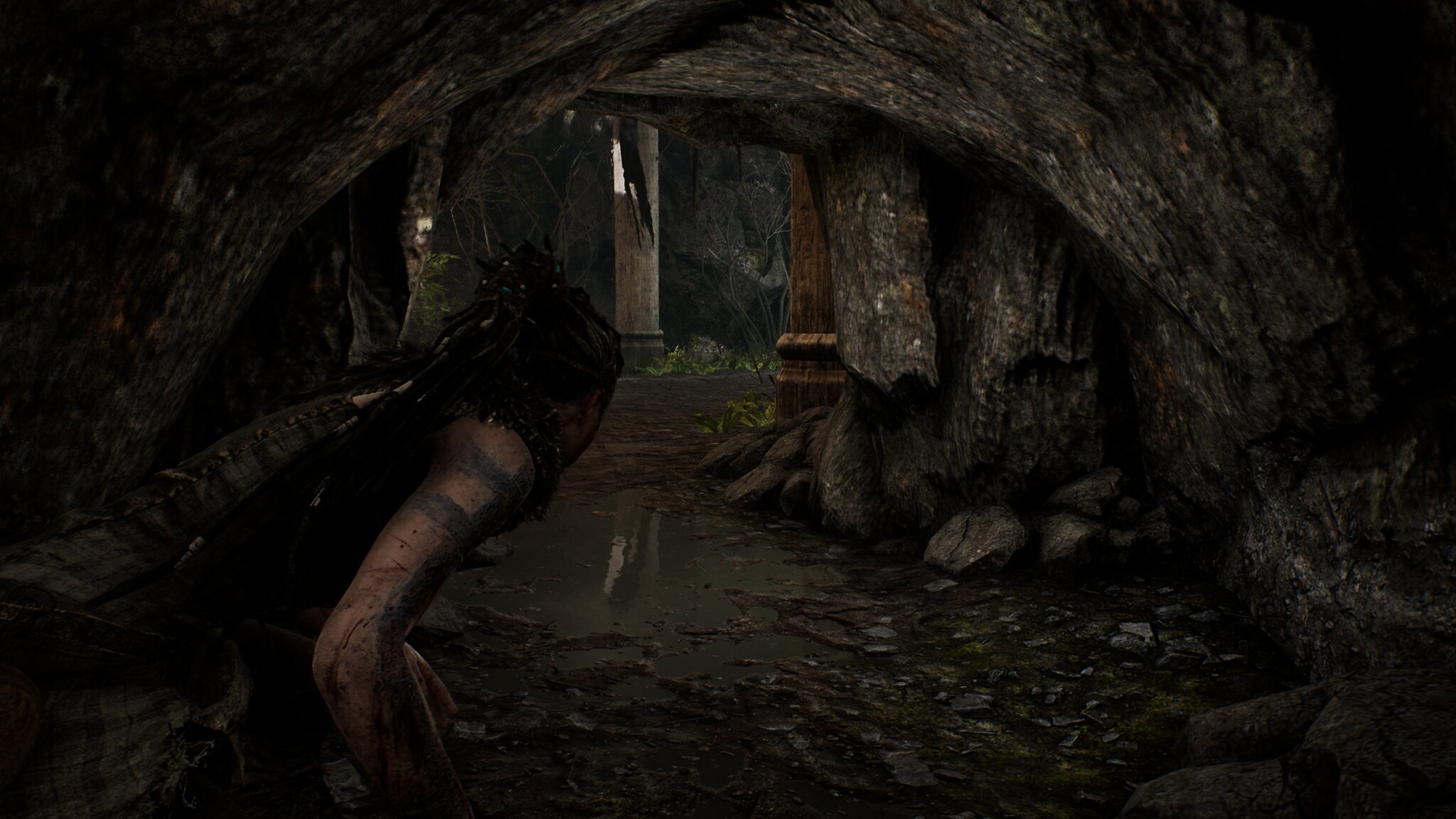The image captures a dark and atmospheric scene from the interior of a cave in a modern video game, with intricate attention to detail. The cave wall is dominated by an ancient, damaged pillar that hints at a forgotten past. The floor is strewn with high-resolution boulders and debris, likely remnants of cave collapses. At the center of the image, slightly off to the left, a lantern fixed to the wall emits a faint glow, struggling to illuminate the surrounding darkness. Multiple light sources penetrate the cavern, casting shadows and adding depth to the rugged landscape. The overall scene is rich in texture and visual cues, showcasing the advanced graphics of contemporary gaming technology.